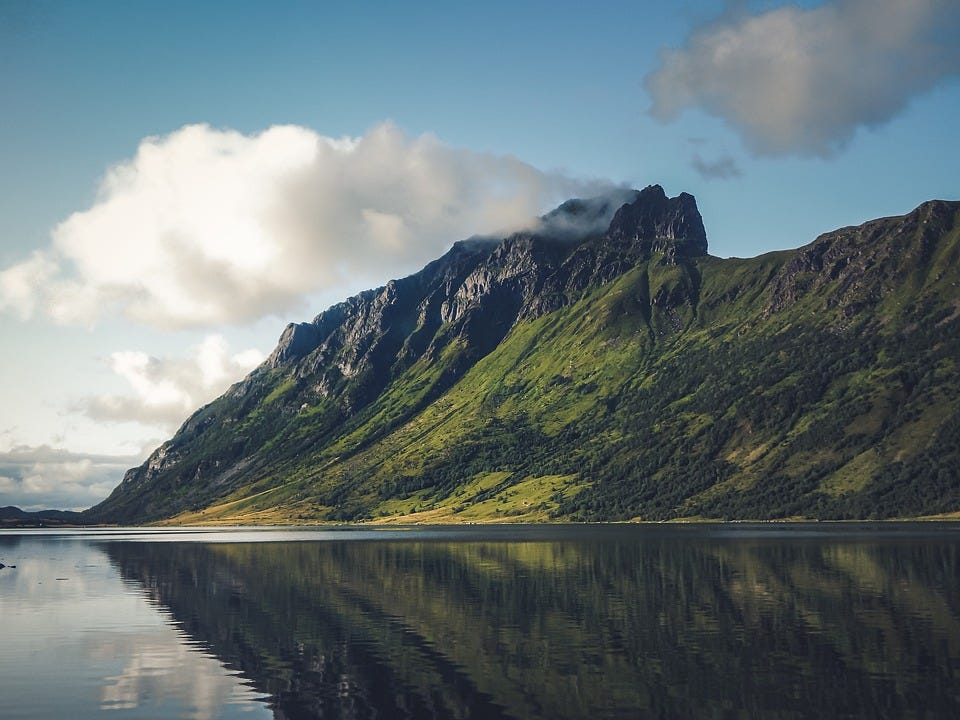This captivating rectangular photograph, taken from a ground-level perspective in the middle of a calm lake, perfectly encapsulates a serene and unspoiled natural landscape. The smooth, glass-like water dominates the bottom third of the image, reflecting the rich scenery above with minimal ripples. Rising majestically at the center is a massive mountain, its slick, rocky cliff glinting under the sunlight. The mountain's lower slopes are adorned with verdant greenery, transitioning into a lush hillside with trees, shrubs, and patches of grass, suggesting a vibrant spring setting. The tranquil scene extends to the upper third of the image, where a partly cloudy blue sky hovers overhead, with fluffy white clouds nestling into the mountain's crevices. Notably, no signs of civilization such as buildings, people, boats, or cars are present, highlighting the pure and untouched beauty of this natural setting.